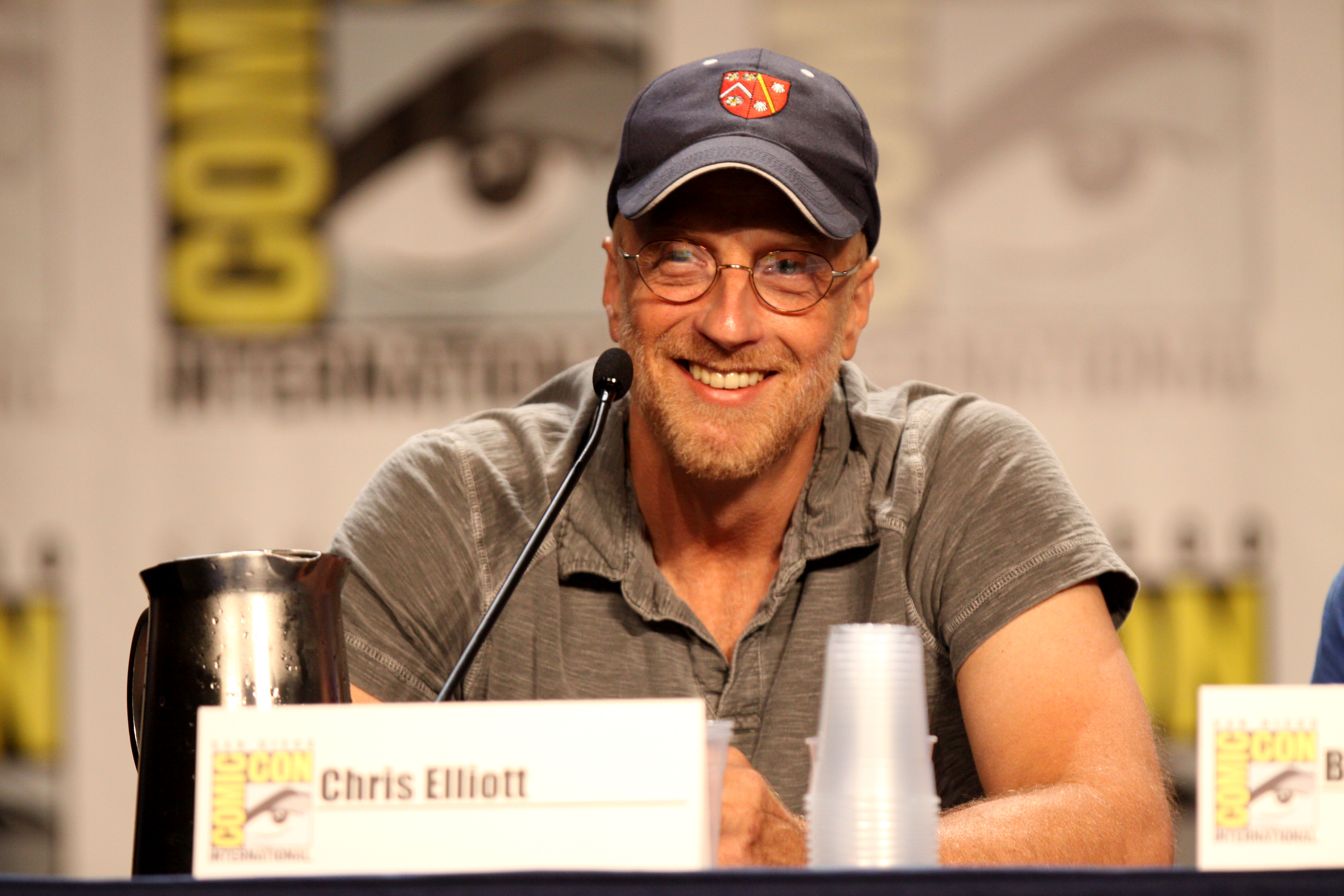The photograph captures a man identified as Chris Elliott sitting at a table draped with a black tablecloth. He is centered in the image and visible from his lower chest up to his head. Chris sports a blue baseball cap adorned with a red shield logo and wears rounded glasses. He has a short light-colored mustache and beard, and his short-sleeve polo shirt, which is a grayish-brown color, has all three buttons undone. 

In front of Chris on the table is a white nametag featuring the Comic-Con logo on the left side, with his name, "Chris Elliott," printed in black text. Positioned directly behind the nametag is a silver pitcher, glistening with droplets of condensation. To its right, a stack of clear plastic cups can be seen. Chris is speaking into a thin black microphone that extends towards him from the left side of the frame. 

The background is blurred but displays a wall covered with multiple Comic-Con emblems, reinforcing the setting of the event. Chris is looking slightly to his left, smiling with his top front teeth visible, adding a friendly and engaging demeanor to the scene.